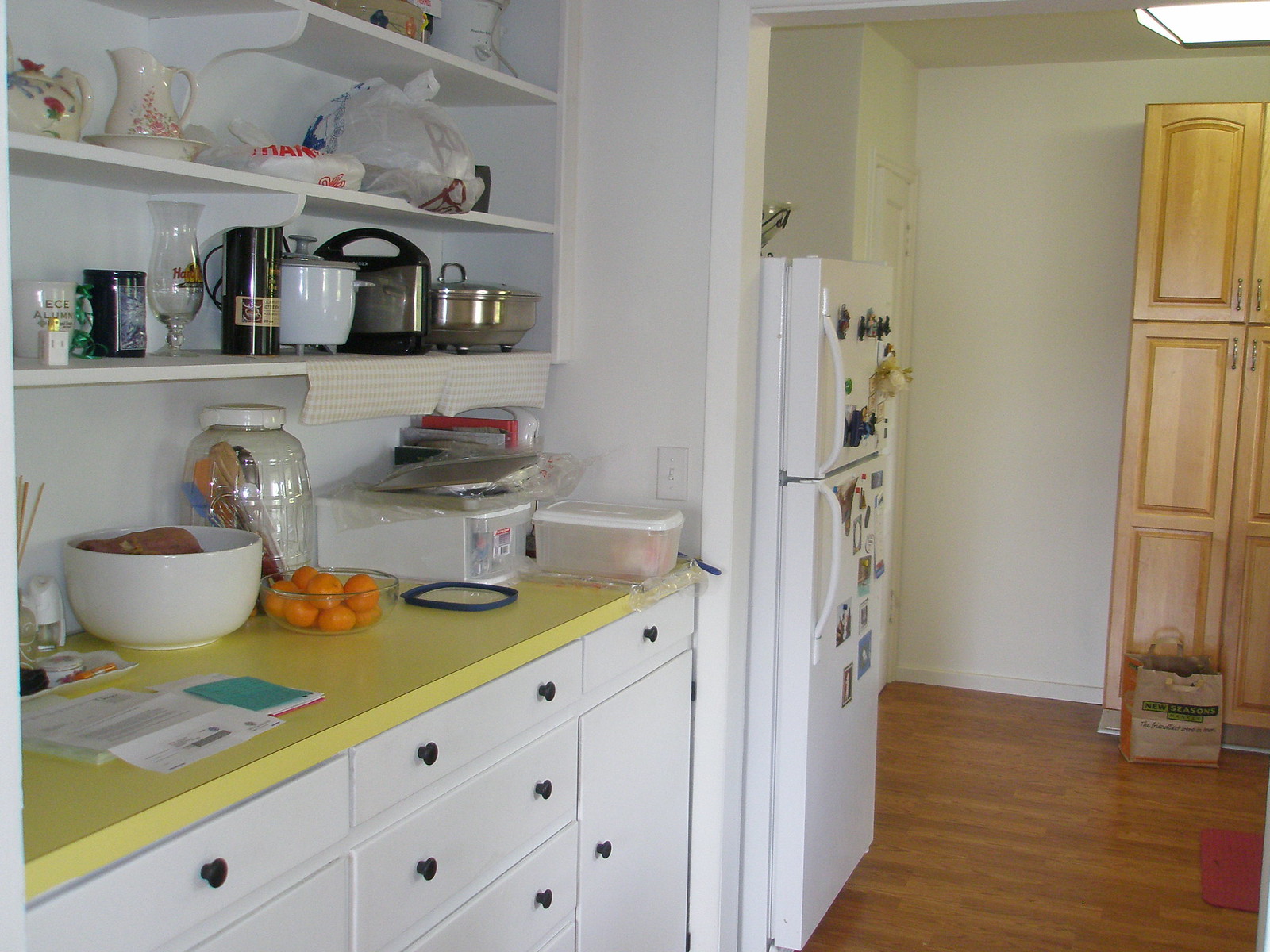This kitchen interior features a harmonious blend of white and wooden elements. The walls are painted in a clean white, providing a bright and airy atmosphere. Against one wall stands a brown pantry adorned with elegant gold knobs, illuminated by a sleek white light fixture above it. A red rug adds a touch of warmth and color on the polished wooden floors.

To the left, a white refrigerator with matching handles is embellished with an assortment of magnets and pictures, offering a personal touch to the space. Atop the fridge sits a vibrant green bowl, adding to the room's color palette. The countertops, fitted with silver knobs, host a variety of kitchen essentials. A Tupperware container filled with items is placed next to a collection of cookbooks on the right. An upside-down blue Tupperware lid lies nearby, possibly set aside after recent use.

A white bowl filled with fresh oranges sits next to a sizeable container holding an array of spoons. The counter also displays an air freshener and a couple of diffusers, alongside an open piece of mail and a green letter, indicating the kitchen is very much a lived-in, functional space. Above this setup, shelves hold a silver pot, a waffle maker, a rice maker, cups, coffee mugs, a large pitcher, and some plastic bags, ensuring that all necessary cookware and items are within easy reach.

Overall, this kitchen exudes a sense of organized chaos, combining functionality with a warm, welcoming ambiance.